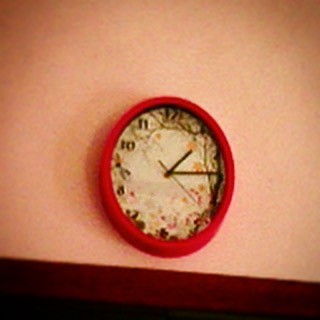This is a square-shaped, color photograph taken indoors under artificial lighting. The image, although low resolution and slightly blurry, features a round, rustic, and somewhat antique-looking clock placed against a peach-colored wall with distressed, sponged-on white and beige splotches. The clock has a distinctive red edge encasing a marbled tan and off-white face embellished with green, pink, and yellow floral designs. The black numerals are partially obscured by the distressed coloring, but the 12, 11, 10, and 8 are visible. The clock's three hands—a short, thick black hour hand, a longer thick black minute hand, and a skinny black second hand—indicate a time of a quarter past two, with the second hand at around the 20-second mark. Slight shadows are cast on the wall, suggesting light coming from the right. Below the clock, a darker wooden area, possibly mahogany or trim, spans the bottom of the photograph, transitioning from a deep red to dark brown towards the bottom left.